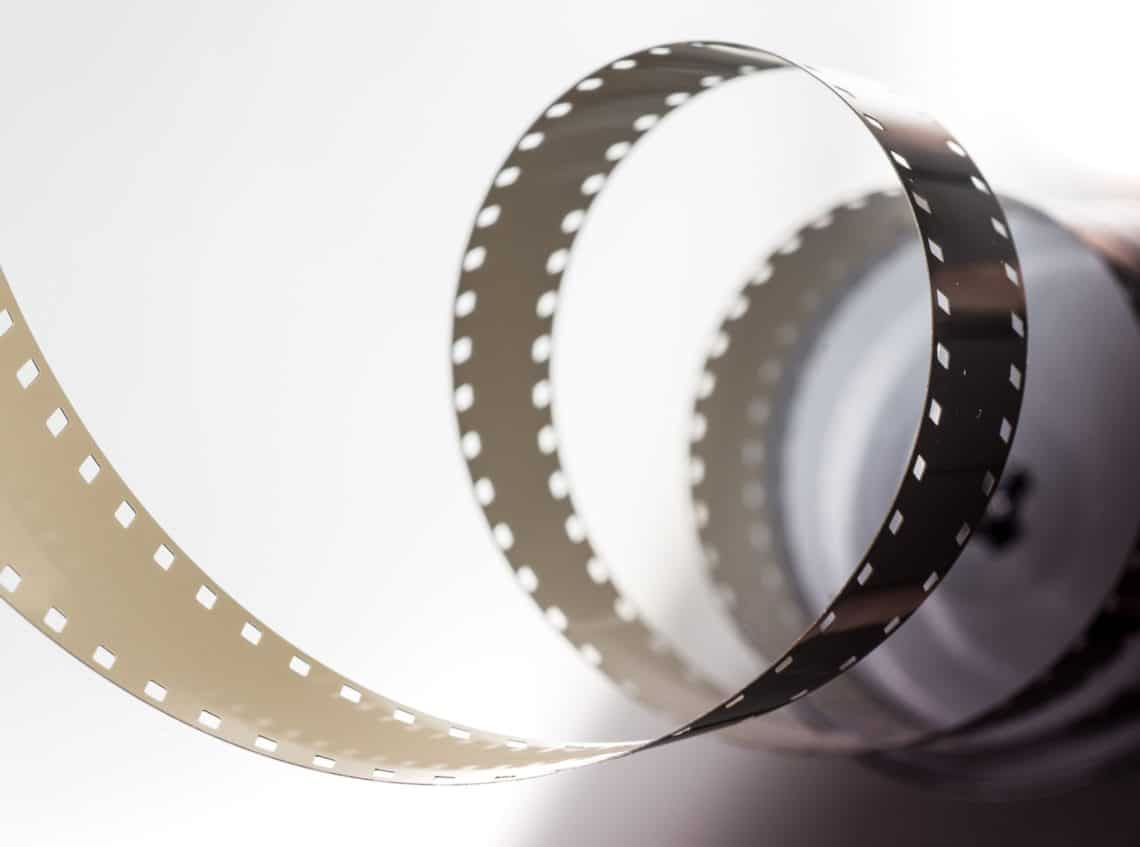This photograph captures a close-up view of a film reel, with a strip of 16 or 35mm movie film partially uncoiled and spiraling from the left to the right against a light gray or white background. The film, which appears to be undeveloped and thus exposed to light, features characteristic square punch-outs along both edges. The strip exhibits a gradient from lighter brown on the inside to darker brown on the exterior. The film loops twice, starting at the bottom left and continuing towards the upper left side. The reel itself, made of silver metal, is visible in the background on the right. The picture is somewhat blurry, especially around the reel, with discernible shadows in the right-hand corner, adding depth to the composition. Overall, the image evokes the nostalgic essence of traditional film projection, reminiscent of old movie theaters or vintage cameras.